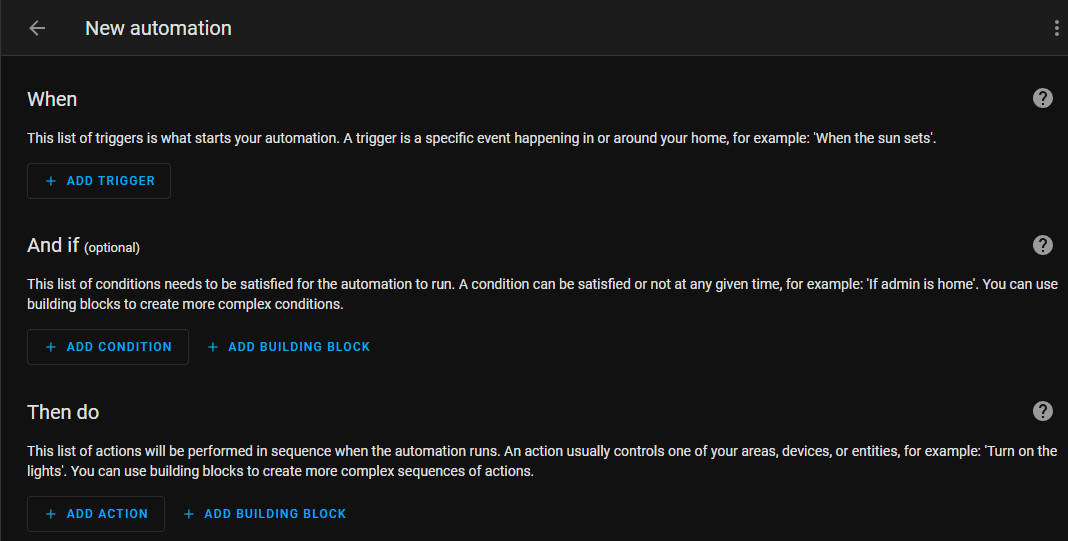**Detailed Caption for the Settings Page Screenshot:**

This screenshot captures a settings page with a visually distinct layout. The top-left corner features a dark grey header. Within this header, a light grey arrow points to the left, followed by white text that reads "New Automation." At the far right of this header, three light grey dots are stacked vertically, indicating additional options.

Below the header, the main body of the page stands out with a black background, divided into three sections:

1. **When Section:**
   - Positioned at the top-left, this section is introduced by bold white text saying "When."
   - Directly beneath "When," smaller text explains its significance: "This list of triggers is what starts your automation. A trigger is a specific event happening in or around your home. For example, when the sun sets."
   - To the upper right of this description, a white circle encloses a black question mark, likely signifying help or additional information.
   - Adjacent and to the left of the text, a black box outlined in thin light grey contains blue all-caps text "ADD TRIGGER," right-justified with a blue plus icon to its left.

2. **And If Section (Optional):**
   - Just beneath the "When" section, black text reads "And If," followed by smaller text in parentheses indicating it's optional.
   - Two lines of white descriptive text clarify: "This list of conditions needs to be satisfied for the automation to run. A condition can be satisfied or not at any given time. For example, if admin is home, you can use building blocks to create more complex conditions."
   - Another white circle with a black question mark icon is located to the upper right of this section, providing consistent help icons throughout.
   - Below this description, two buttons aligned to the left are available:
     - The first button, designed similarly to the one in the "When" section, reads "ADD CONDITION" with a plus icon.
     - The second button, also in a similar style but without an outline, reads "ADD BUILDING BLOCK" accompanied by a plus icon to its left.

The overall design is sleek, utilizing a dark background with light-colored text and icons to ensure readability and user clarity.